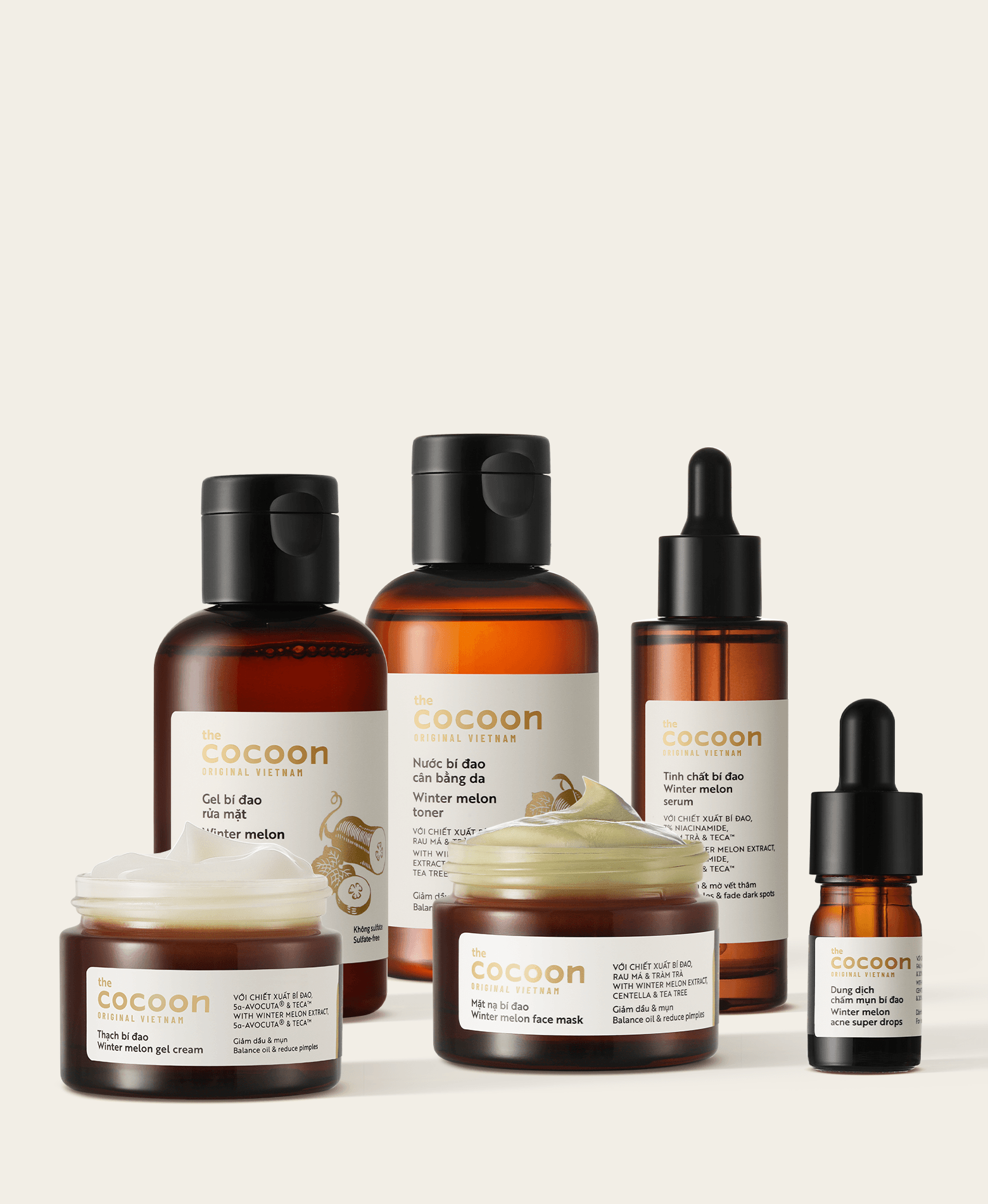This indoor photograph, styled like an advertisement, showcases six skincare products from the brand Cocoon. They are neatly arranged on a light gray surface that matches the background. The central focus is a prominent, wide, short bottle with orange-toned liquid, topped with a black cap, labeled "Cocoon Original Vietnam Winter Melon Toner." Flanking this centerpiece to its left is a similar bottle with a slightly amber liquid, also labeled "Winter Melon" though the word "toner" is partially cut-off. Further left is an opened, dark brown bottle uncovering a "Winter Melon Gel Cream." To the right of the main bottle stands another resembling the leftmost one, tagged "Winter Melon Face Mask," followed by a small, jar-like container with a black top, labeled "Winter Melon Acne Super Drops." The final item, positioned on the far right, is a narrow bottle with a dropper top, labeled "Winter Melon Serum." All products bear a uniform white label with gold "Cocoon" branding and text in both Vietnamese and English, emphasizing their original Vietnamese heritage.